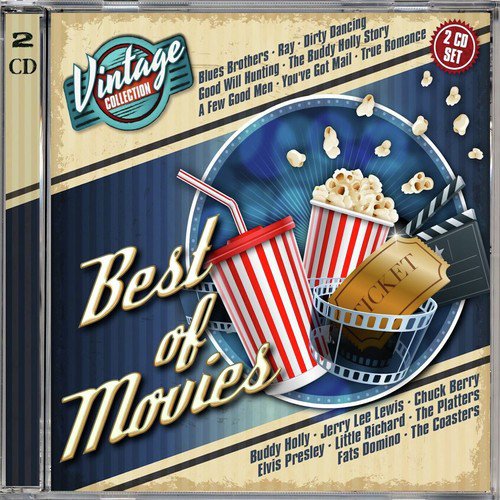This square-shaped image depicts the front cover of a CD album case, prominently showcasing a "Best of Movies" collection. The background is a light tan color, with a navy blue ribbon diagonally spanning from the bottom left to the top right. This ribbon intermittently features various text, such as "Best of Movies" and a logo that reads "Vintage Collection." 

In the upper left-hand corner is a circular red label stating "Two CD Set." Additionally, a similarly styled blue circle indicating "Vintage Collection" can be found on the left side. The center of the cover displays a nostalgic movie-themed design with a red and white striped popcorn bucket bursting with popcorn, a matching red and white soda cup complete with a straw and red cap, a strip of film, and a golden movie ticket.

The names of various artists and iconic movies feature across the cover, both at the top and bottom. The top lists: "Blues Brothers, Ray, Dirty Dancing, Good Will Hunting, The Buddy Holly Story, A Few Good Men, You've Got Mail, and True Romance." Below the central illustration, the artists included are "Buddy Holly, Jerry Lee Lewis, Chuck Berry, Elvis Presley, Little Richard, The Platters, Fats Domino, and The Coasters."